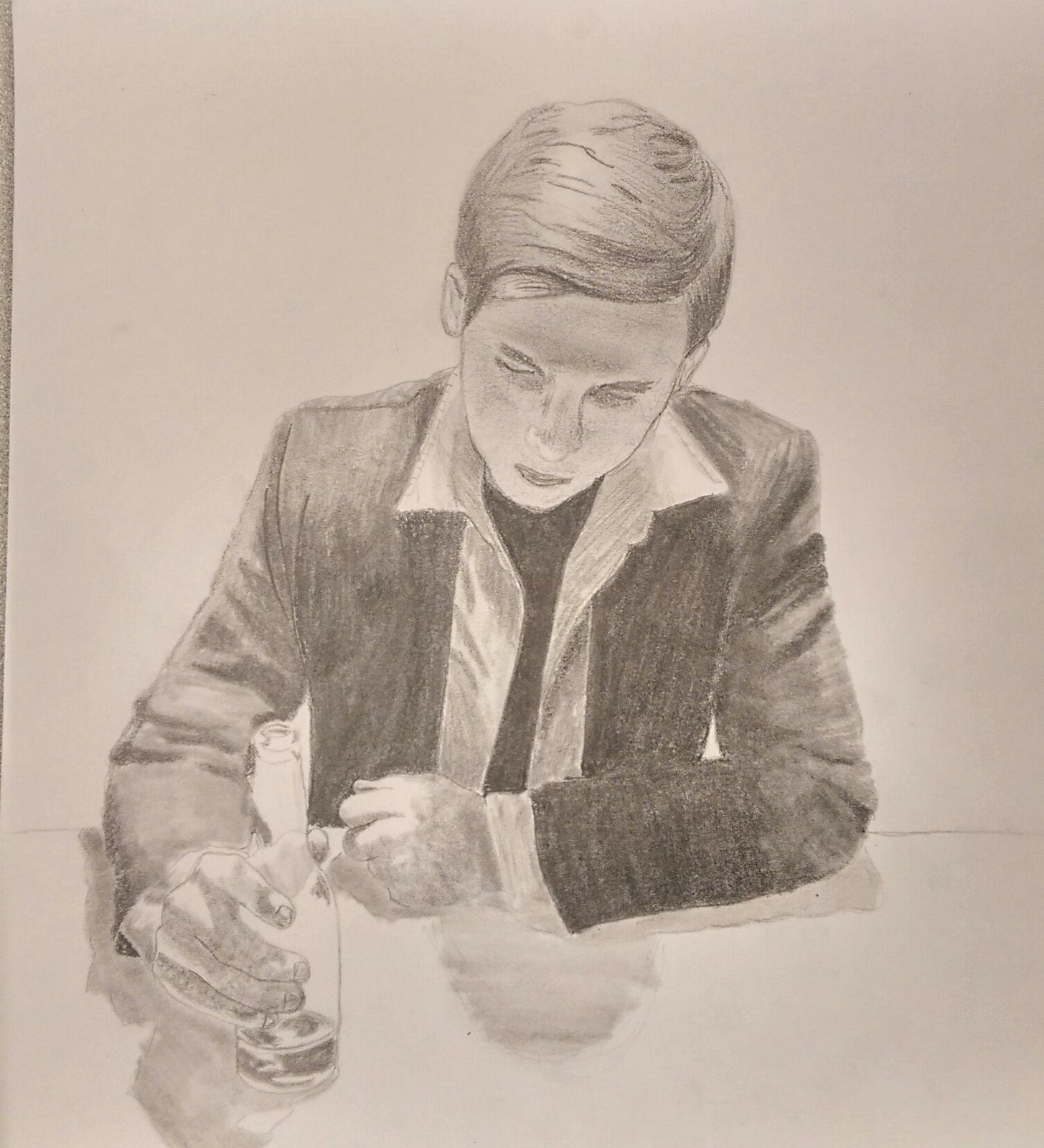The image is a meticulously detailed pencil sketch depicting a young man, likely between the ages of 18 to 20, dozing off at a bar. He wears a black dress jacket over a black undershirt and a white collared work shirt. His short, brown hair is combed to the left, and his eyes are closed as he rests his head forward, with his left arm bracing him on the table. The right arm extends downward, clutching an almost empty, older-style Budweiser bottle, with about 20% of the dark liquid visible at the bottom. The background remains unfilled with pure white, accentuating the detailed shading on the figure. Shadows accentuate the contours of his hands and arms, and there's a hint of erased or scratched marks under his left arm. Despite the sketch's unfinished background, the composition is rich with texture and depth, offering a striking monochromatic portrayal of fatigue and contemplation.